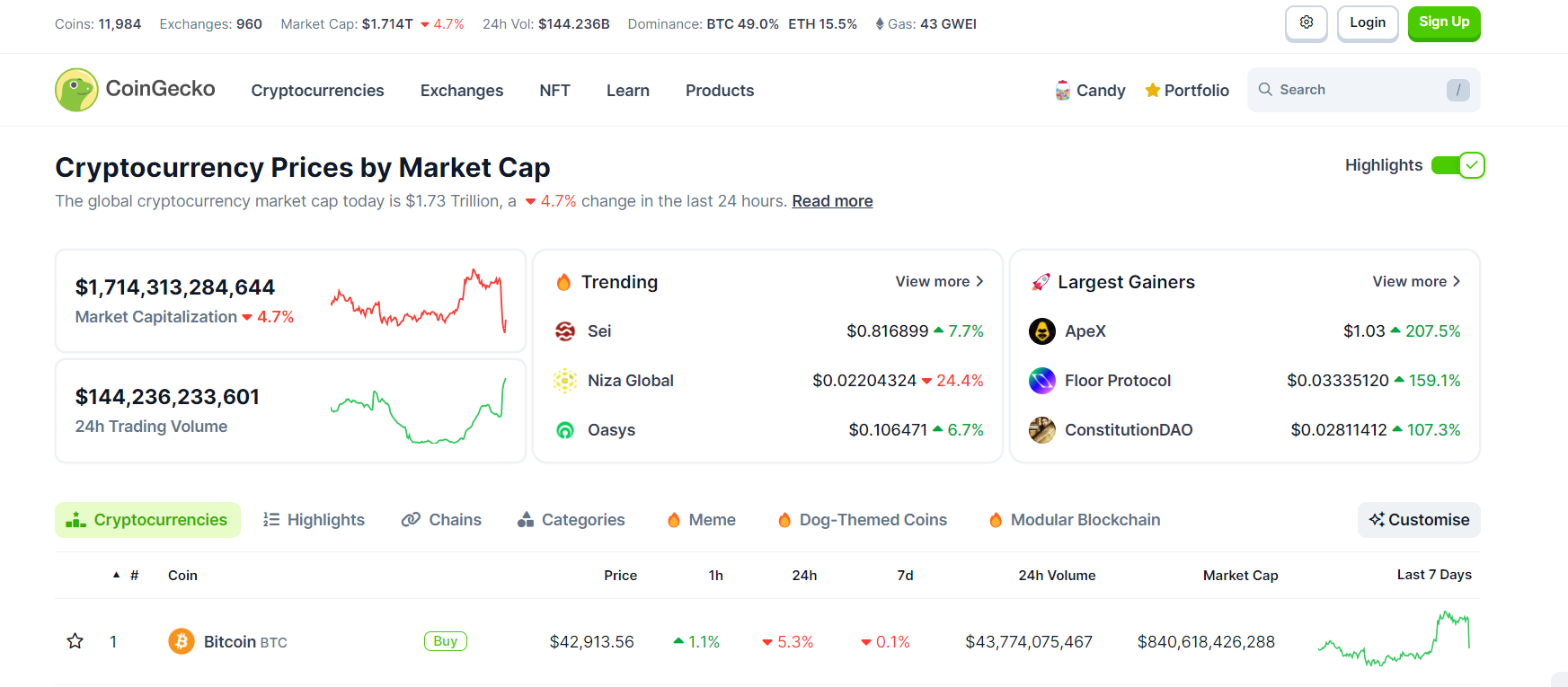The screenshot depicts the homepage of CoinGecko, a cryptocurrency market tracking website. Prominently displayed on the left is the CoinGecko logo, featuring an adorable green gecko encircled by a yellow ring. To the right of the logo, a navigation menu includes options such as 'Cryptocurrencies,' 'Exchanges,' 'NFT,' 'Learn,' and 'Products.'

Above the main content, vital ticker information is presented, detailing:
- Total coins: 11,984
- Total exchanges: 960
- Market cap: $1.714 trillion (down 4.7%)
- 24-hour volume: $144.236 billion
- Market dominance: Bitcoin (BTC) at 49% and Ethereum (ETH) at 15.5%
- Gas fees: $43 GWEI

On the upper right side of the interface, there are a settings button represented by a gear icon, a white 'Login' button, and a green 'Sign Up' button.

Below these, the page features illustrative charts depicting market capitalization and 24-hour trading volume. The market capitalization chart, rendered in red, indicates a downward trend, while the trading volume chart, in green, shows an upward trend.

Highlighted within the interface are trending cryptocurrencies such as SEI, NISA Global, and Oasis. Additionally, notable gainers include Apex, Floor Protocol, and Constitution DAO.